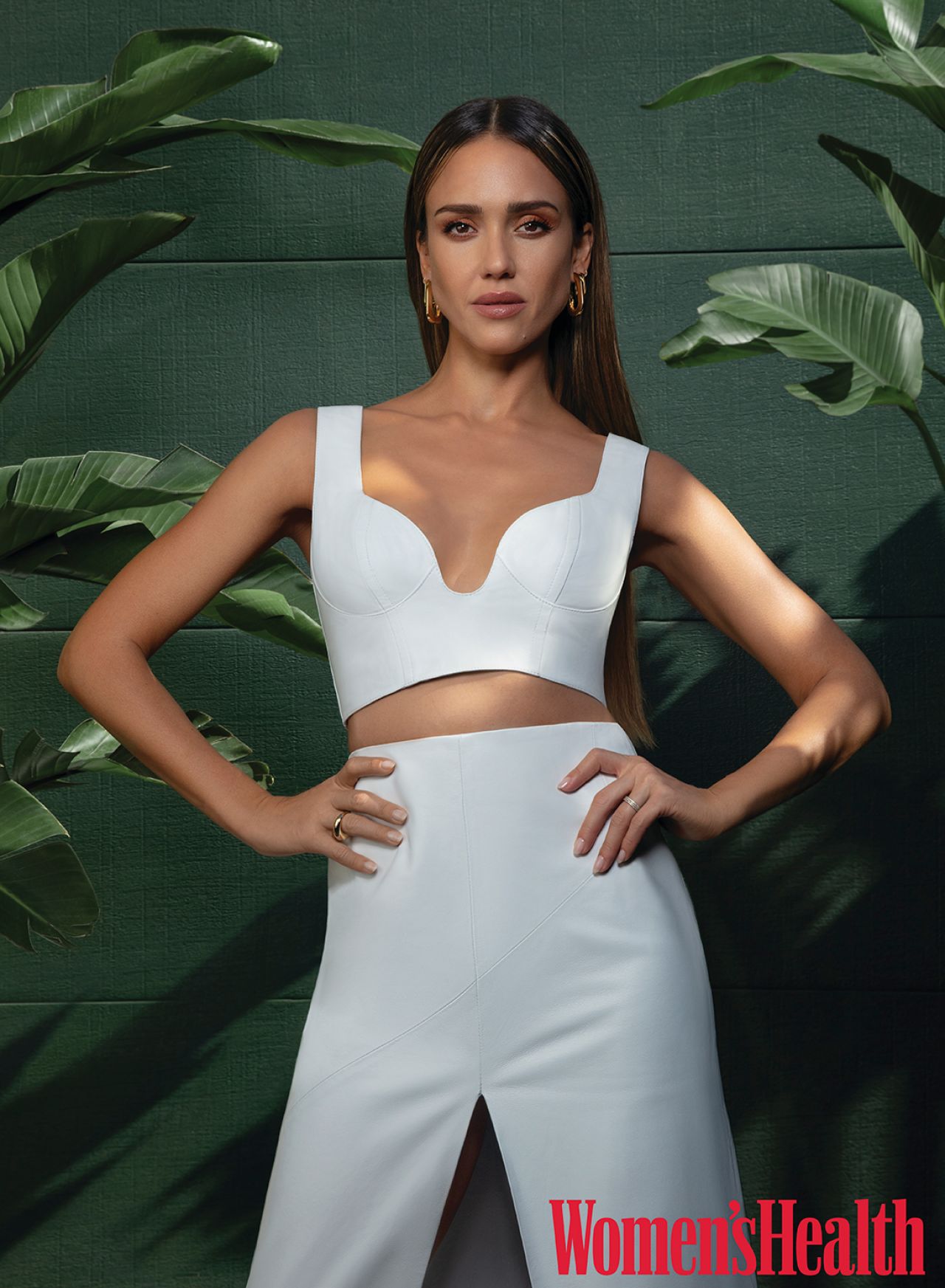The image is a high-resolution, portrait-mode magazine cover featuring what looks like Jessica Alba standing in a powerful yet fashionable pose, typical of a Women's Health Magazine cover—indicated by the red text at the bottom right. She is dressed in a modern, all-white outfit consisting of high-waisted, plasticky pants that reach her navel, and a matching white crop top that reveals her midsection, presenting a summery and somewhat futuristic look. Jessica Alba, a youthful, olive-skinned woman with long, straight dark hair slicked back, adorns gold hoop earrings and a large gold ring with a prominent diamond on one of her fingers. Her eye makeup appears to have a reddish hue. She stands confidently with her hands on her hips, set against a green-painted wooden wall with visible slats and shadowy tropical palm leaves behind her, enhancing the overall tropical, vibrant theme.